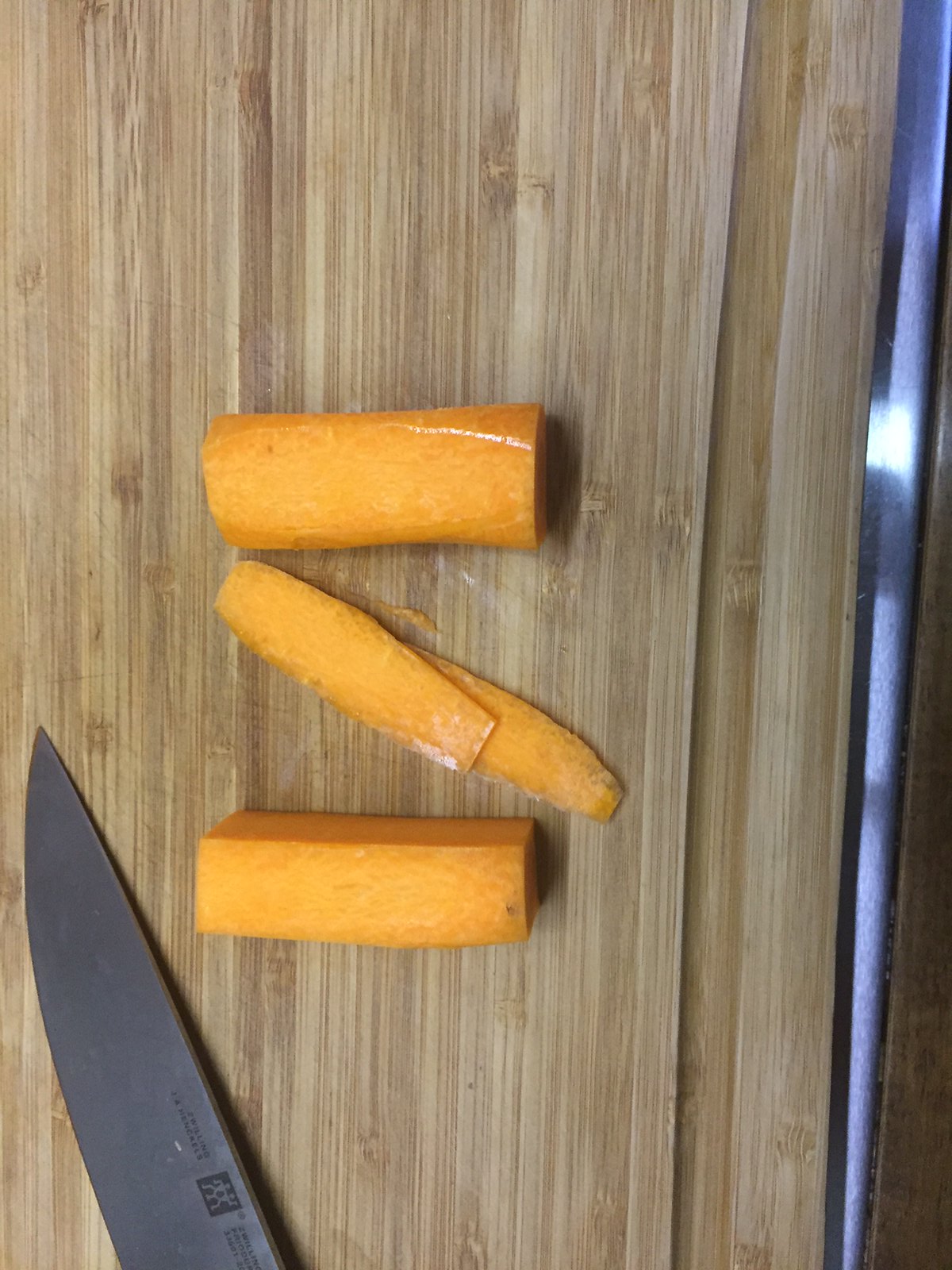This vertically rectangular image captures a wooden cutting board with a light-colored grain running vertically from top to bottom. Dominating the right side of the image is a mysterious blue band that resembles a light, possibly suggesting a view into another room. On the bottom left-hand corner, the blade of a knife is visible, its black metal contrasting sharply with the wood, with the tip pointing upward. In the center of the cutting board are four pieces of what appears to be carrot, though they could also be yams due to their yellowish-orange hue. The bottom piece is a squared chunk, followed by two thin slices that lie on top of each other, resembling peels. Above those, there is a slightly elongated, cuboid piece with its ends neatly cut off, indicating precision slicing. The arrangement of these elements suggests a scene just after some vegetable preparation.